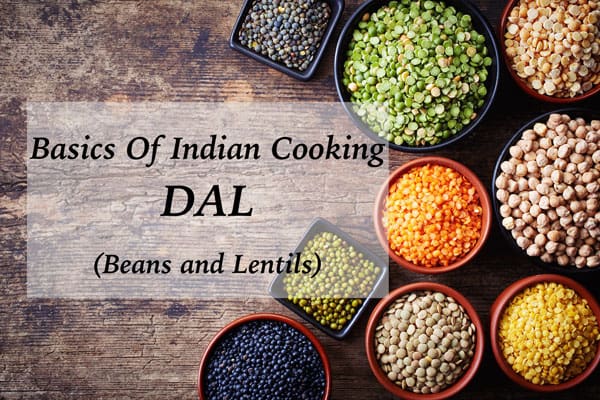The detailed color photograph captures an assortment of dried beans and lentils, characteristic of Indian cooking, arrayed within nine bowls against a rich, brown wooden table. Predominantly positioned to the right and bottom center of the image, the bowls vary in shape and color, featuring black and square designs. From top right to bottom left, the bowls exhibit an array of beans and lentils: beige lentils, chickpeas, yellow corn, and tan chickpeas, alongside vibrant orange and green lentils. The image also includes an opaque white rectangle on the left side, overlaid with black text stating "Basics of Indian Cooking" with "D-A-L" prominently centered below, followed by "(beans and lentils)" in parentheses. The photograph merges realism with graphic typography, presenting a visually engaging entry into the essentials of Indian culinary ingredients.